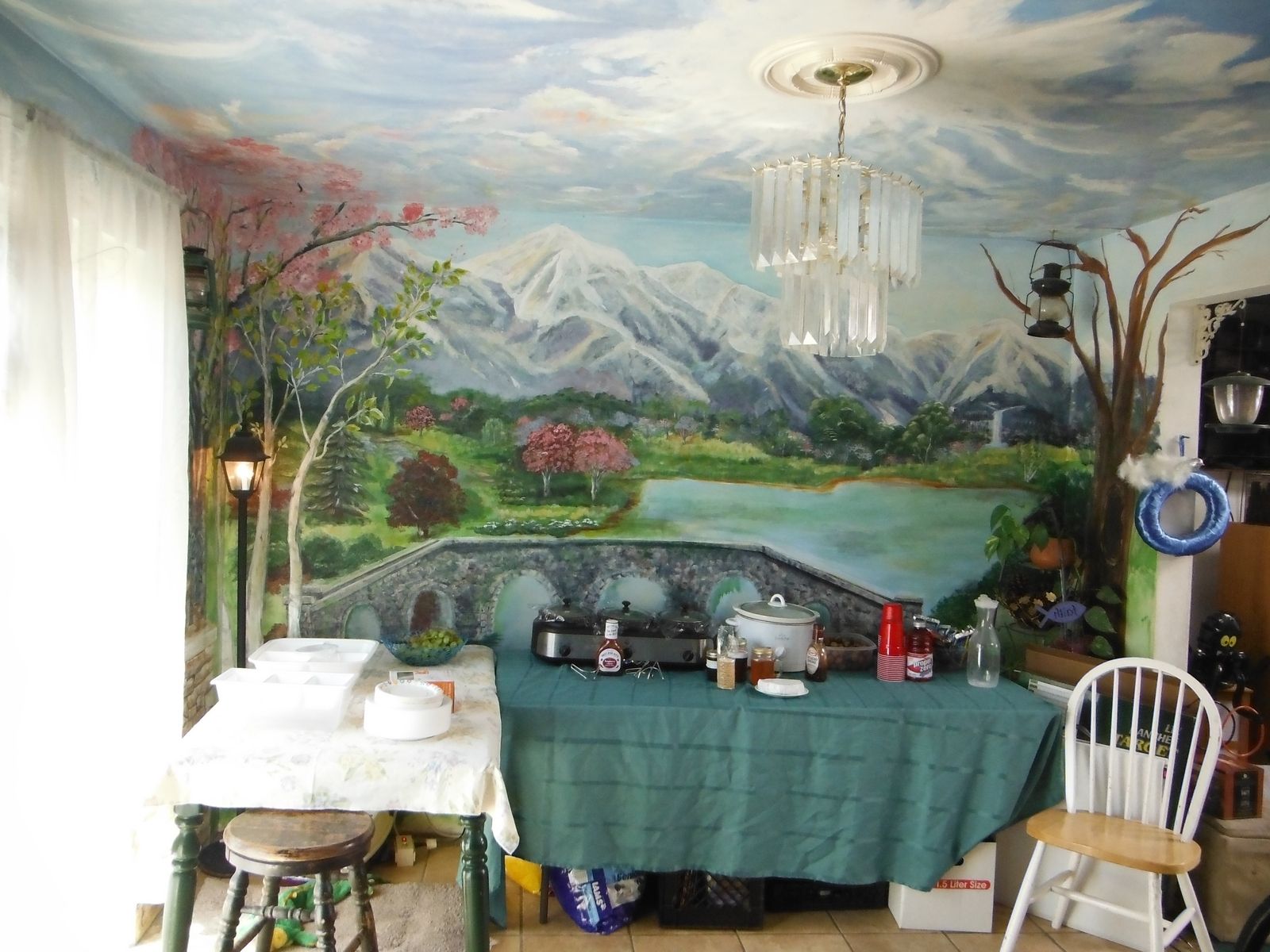The image depicts a detailed indoor scene of a room in a house adorned with a continuous, immersive mural that spans the walls and ceiling. The mural showcases a lush, green valley nestled amid snow-capped mountain peaks, complete with a serene lake surrounded by trees, including evergreens and pink flowering varieties. A distinctive rock bridge with three arches traverses the water, adding a rustic charm. Extending onto the ceiling, the mural morphs into a vibrant sky filled with blue hues and white clouds. The central focal point of the ceiling is a crystal chandelier that adds an elegant touch.

Upon the wooden floor, there are two folding tables arranged perpendicularly. One table, covered with a green blanket, is placed prominently in the center and holds various items including a crockpot, a three-section warmer, a barbecue sauce bottle, and red Solo cups. The adjacent table, draped with a white tablecloth, exhibits styrofoam takeout trays, plates, and a glass full of green grapes. Additional elements such as a white farm chair, a wooden stool, and boxes are scattered around.

On the left wall, there is a large window dressed with a lace curtain, while the right wall features a squared arch doorway adorned with two blue wreaths. An intricate lantern hangs in the upper right corner, contributing to the room's rustic yet cozy atmosphere.